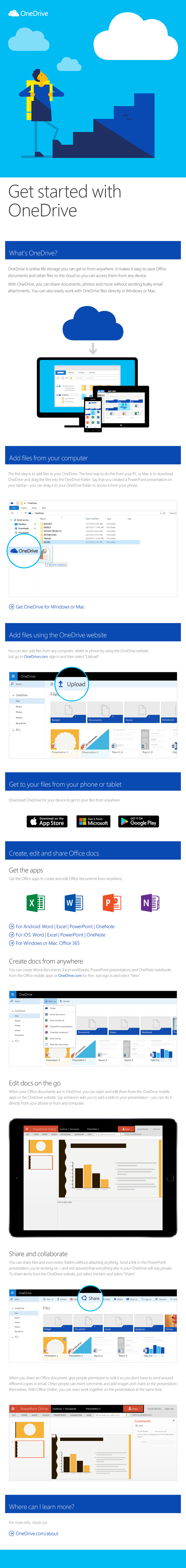The image portrays a section of a website with a predominantly blue color scheme, centered on the Microsoft OneDrive service. At the top of the page, there is a medium bright sky blue background adorned with two overlapping clouds. The text "OneDrive" is prominently displayed, with capitalized 'O' and 'D', against this backdrop.

Beneath this, the background transitions into a lighter blue cloud, complemented by a larger white cloud on the right. A cartoon character is depicted ascending a set of cartoon steps. Below this illustration, the phrase "Get Started with OneDrive" is prominently featured.

Next, a darker blue banner with the text "What's OneDrive?" descends from the top, providing an explanation about the service. An icon of a cloud with a downward arrow pointing towards a computer monitor is shown, along with representations of a tablet and a cell phone.

Further down, another blue banner is labeled "Add Files from Your Computer," explaining the process of uploading files. This section features a white background with an illustration of files being dropped down and the OneDrive logo, which consists of a cloud next to the text "OneDrive" enclosed in a blue circle. This part encourages users to "Get OneDrive for Windows or Mac."

Additionally, another blue banner with the text "Add Files Using the OneDrive Website" offers further instructions. Finally, there is a black banner featuring the OneDrive logo once more, alongside a highlighted section that reads "Upload," accompanied by an upward arrow above a line, signifying the upload functionality.